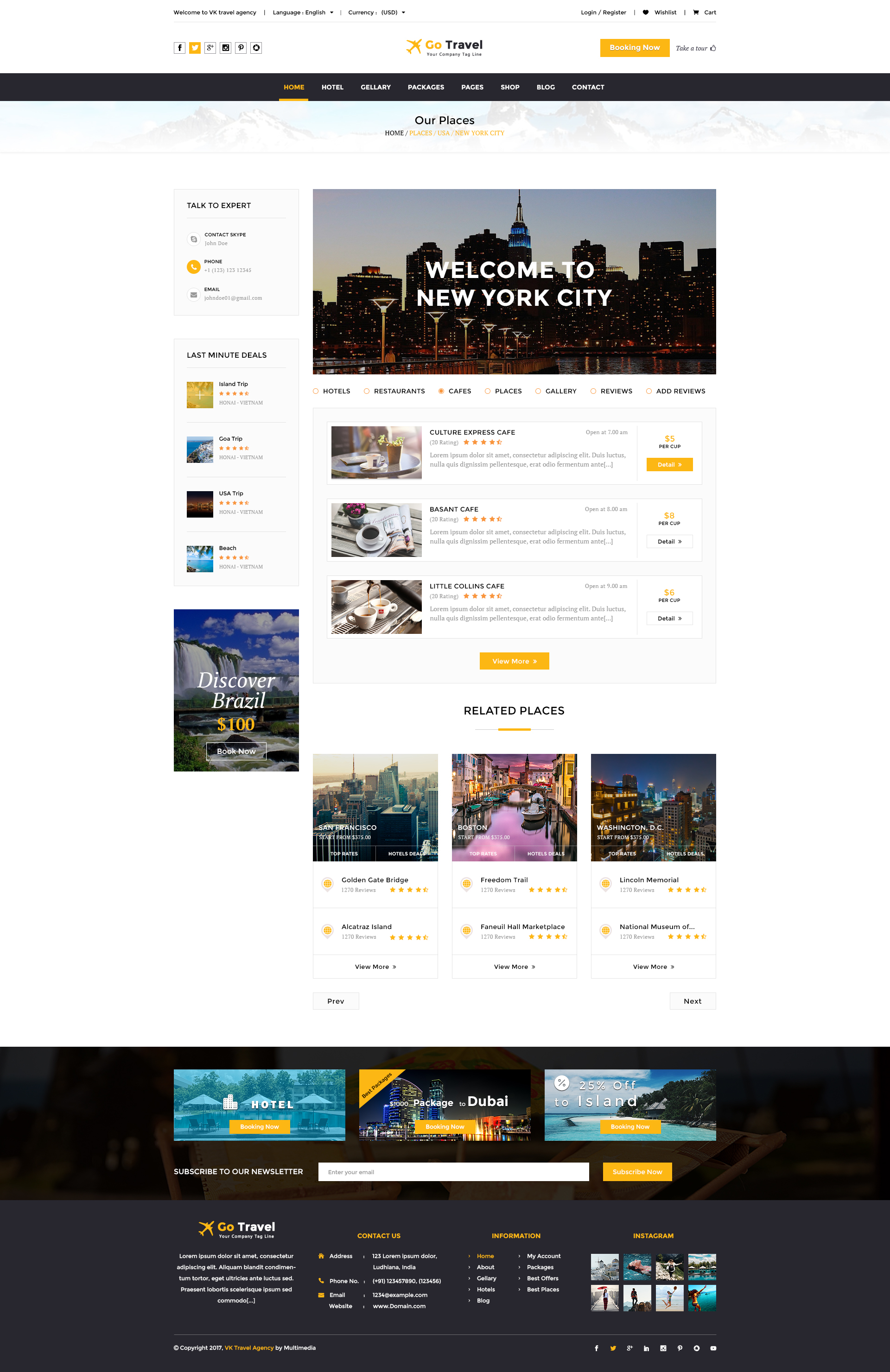Here is a cleaned-up and detailed caption for the image:

---

This screenshot features a travel website. At the top of the image, a white navigation bar showcases a logo on the left: a yellow airplane icon followed by the word "go" in yellow font and "travel" in black font. Accompanying the logo, social media icons for Twitter, Facebook, Instagram, Pinterest, and Google are aligned to the left. On the right side of the bar is a yellow button, though the text on it is unreadable. 

Directly beneath the white bar is a black navigation menu with clickable options, including "Home," "Hotel," "Luxury," and "Contact," among others that are hard to discern. Below this menu, the text "Our Places" appears in black font. Dominating the center is an evocative photograph of the New York City skyline at night, overlaid with the welcoming text "Welcome to New York City" in white font.

Further down, the page features numerous travel destination entries which are too small to read distinctly. Following these entries are additional images, including an advertisement promoting travel to Brazil with a highlighted price of $100. The very bottom of the page provides a sitemap with clickable links to various sections of the website.